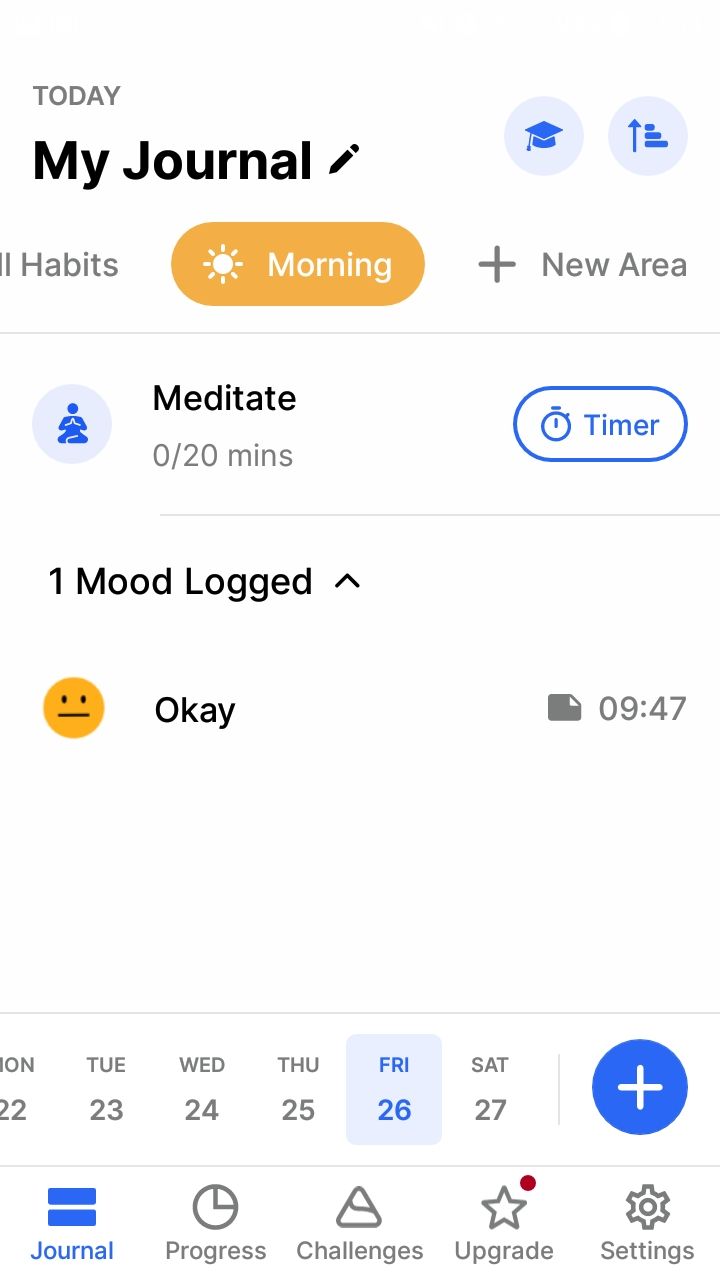The image is a screenshot from a website with an all-white background. At the top of the webpage, the word "TODAY" is displayed in smaller, capitalized print. Below that, in larger print with capitalized letters, is the title "My Journal," accompanied by a pencil icon. 

To the right of this title, there are two blue circles each containing a darker blue graphic. The first circle features a graduation cap, while the second has an arrow pointing upwards next to three lines of varying lengths (small, medium, and long). 

Below the title "My Journal," the word "Habits" is displayed. Beneath this, a yellow-orange banner labeled "Morning" includes a sun icon. Next to this banner, a plus sign signifies an option to add a new area.

Further down, there's a blue circle showing a person meditating with the caption "Meditate: 0 of 20 minutes," along with an option to start a timer. Below it, there's an entry noting "1 mood logged," represented by a yellow smiley face with a neutral expression (a straight line for the mouth and two small eyes), indicating an "Okay" mood logged at 9:47 AM.

A list of days follows: "Monday 22nd," "Tuesday 23rd," "Wednesday 24th," "Thursday 25th," "Friday 26th," "Saturday 27th," with "Friday" being highlighted.

At the bottom of the screenshot, navigation options are listed: "Journal," "Progress," "Challenges," "Upgraded," and "Settings," with a blue circle containing a plus sign nearby.